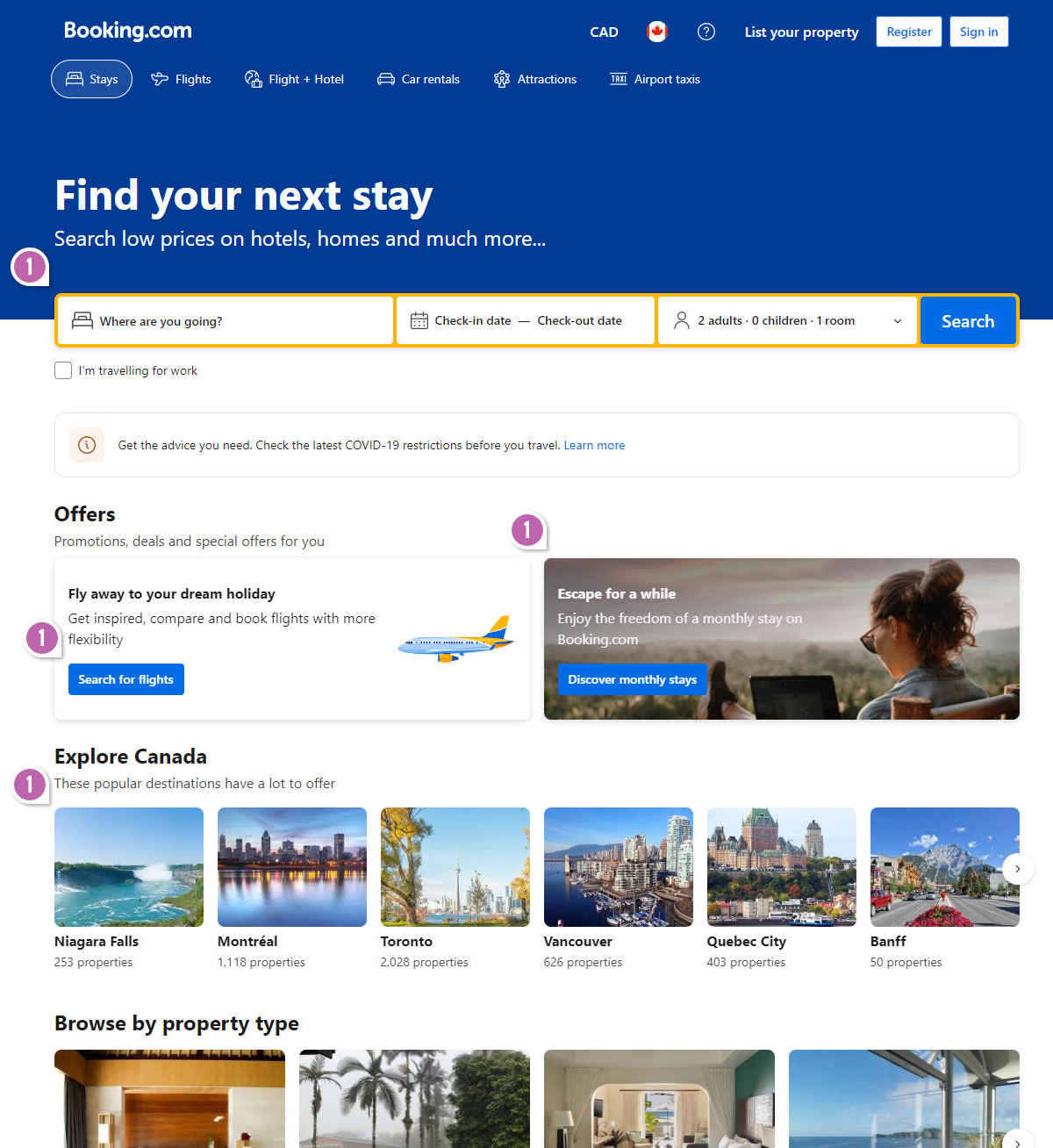The printout from booking.com features a well-organized layout for planning travel. At the top, there's a prominent blue banner with several navigational options: "Stays," "Flights," "Flight + Hotel," "Car Rentals," "Attractions," and "Airport Taxis." To the right, various icons and options are displayed, including "CAD" (Canadian Dollar), "List your property," "Register," and "Sign In," all set in white text against the blue background.

Just below this banner, the text "Find your next stay" is bolded in white, followed by the phrase "Search low prices on hotels, homes, and much more." Beneath this, the search criteria area is highlighted in yellow, allowing users to input details such as destination, check-in and check-out dates, and the number of adults, children, and rooms required. A prominent blue "Search" button is also included.

Further down, a checkbox for "I'm traveling for work" is available. Below this, there's a note saying, "Get the advice you need," encouraging travelers to "check the latest COVID-19 restrictions before you travel," with "Learn more" highlighted in blue for further information.

The document also features blurred clickable options, and photographs of popular Canadian destinations such as Niagara Falls, Montreal, Toronto, Vancouver, Quebec City, and Banff. Additionally, there's a "Browse by property type" section offering various accommodation options for users.